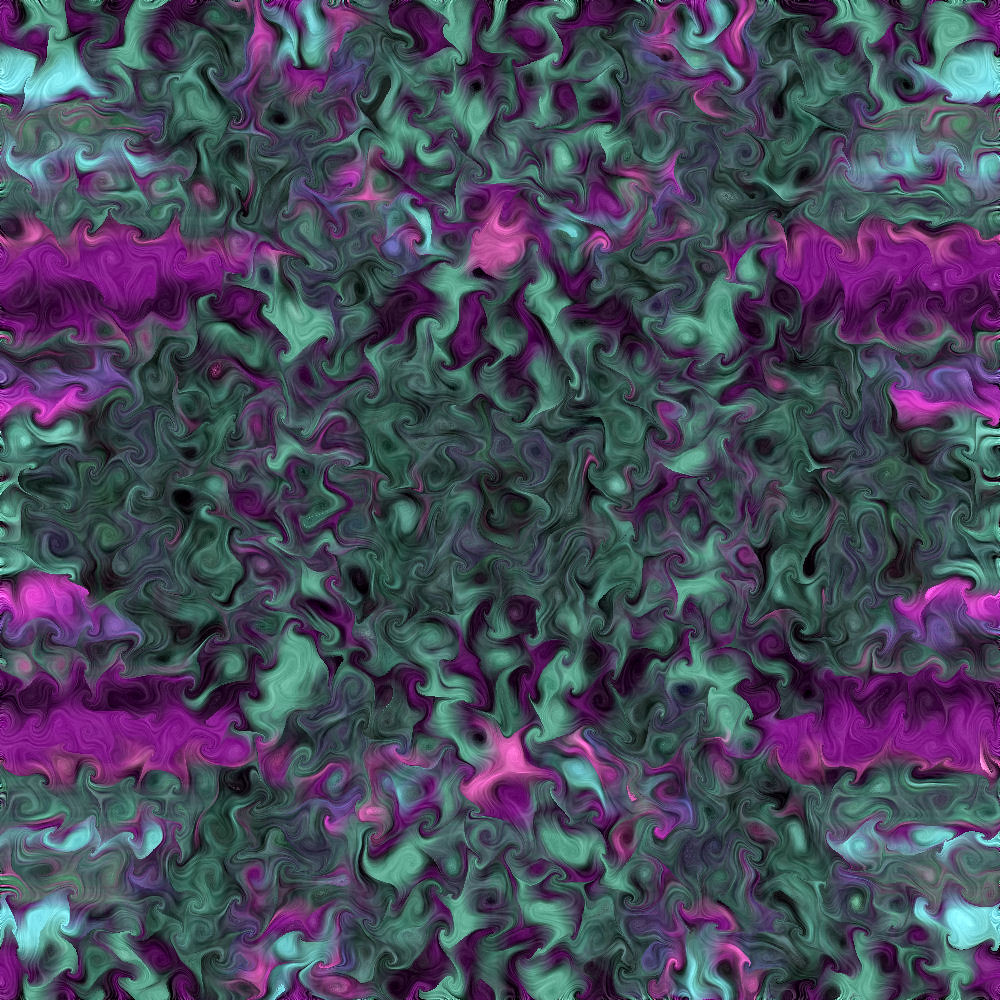This is a close-up photograph of an abstract artwork characterized by a busy, intricate mixture of colors and swirling patterns. The dominant colors are a light green and teal, prominently featured in the center and corners, interwoven with vibrant pinks and purples. Black accents add depth to the composition, which resembles crinkled ribbons or wavy lines compressed together. The piece exhibits a smudged, twirly texture, giving the impression of streaks and twirls made by live paint manipulated with a finger. While the artist’s name and the date are not visible, the detailed and dynamic nature of the painting commands attention, despite the lack of discernible form or recognizable elements.